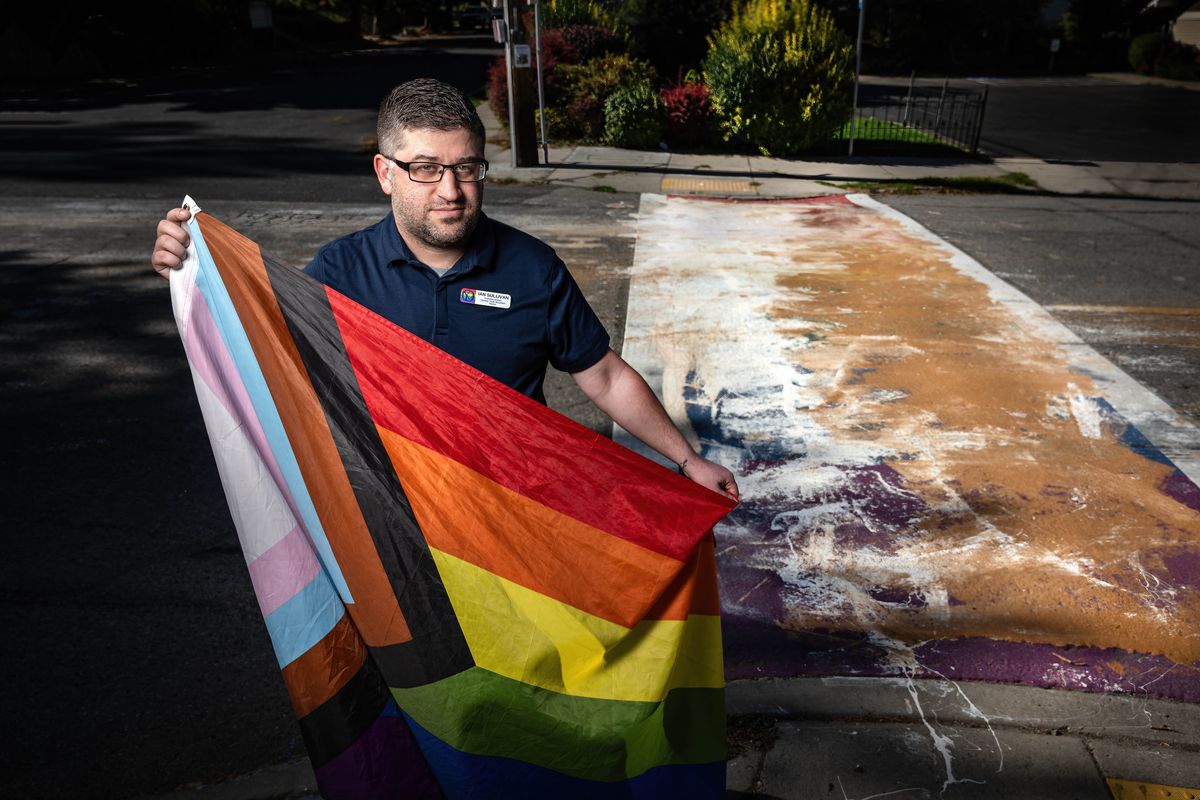This photograph features a Caucasian man wearing a dark blue short-sleeved shirt with a name tag on his top left breast pocket. He has short black hair, cropped shorter on the sides, and a light beard and mustache. The man is also wearing square glasses and stares directly at the camera. He holds the Progress LGBT flag, which includes rainbow stripes (red, orange, yellow, green, blue) on the right and a triangle on the left with black, brown, light blue, purple, and pink stripes, representing a broader spectrum of the LGBT community. 

The man stands on a street, in front of a vandalized crosswalk that appears to have originally been painted with rainbow colors but has been smeared over haphazardly with white and brown paint. The background includes a bush, a fence, and a potential building, with part of the scene shaded in black at the bottom left. The image captures a sense of resilience and support for the LGBT community, as implied by the man's stance and the flag he holds amidst the defaced crosswalk. The photo appears to have been taken during the daytime, adding to the clarity and detail of the scene.